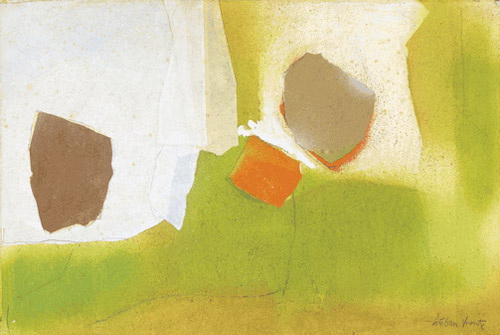This abstract, modern painting features a distinct composition of colors and floating shapes with a minimalist palette. The artwork is divided into two main sections: the lower third is dominated by a base of burnt yellow and green hues. Above this area, the background is primarily white, blending slightly into the green region below. Within the white upper portion, several abstract shapes are suspended in the air. A prominent floating rock-like shape appears in brown on the left side, and nearby to its right is a square-shaped piece in orange. Above these, a misshapen piece with undefined contours floats, primarily white with orange edges at the bottom. The artist's name is discreetly inscribed in small, nearly unreadable letters in the bottom right corner of the painting.